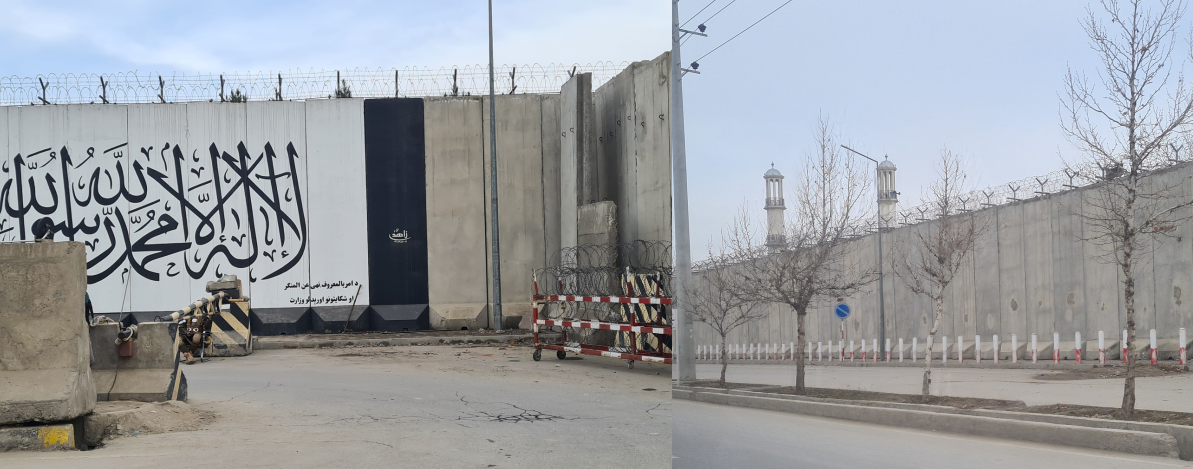The photograph depicts two side-by-side images of high cement security barriers, indicative of a prison or fortified building. Both images prominently feature tall, gray concrete walls topped with razor and barbed wire. The wall on the left reveals dark blue and black graffiti, possibly resembling Arabic writing, against a mostly white and beige background. On either side of the walls are barren trees with no leaves, contributing to the desolate atmosphere. To the right, the second image mirrors the first with similar concrete barriers capped with white fencing and topped with barbed wire, but adds detail with narrow towers and a tall telephone or power line post casting cables overhead. The area in front of these imposing walls consists of cement barriers and a grayish-beige road with visible roadblocks marked by red and white stripes. The background includes a light blue sky, adding a stark contrast to the otherwise muted, industrial setting.